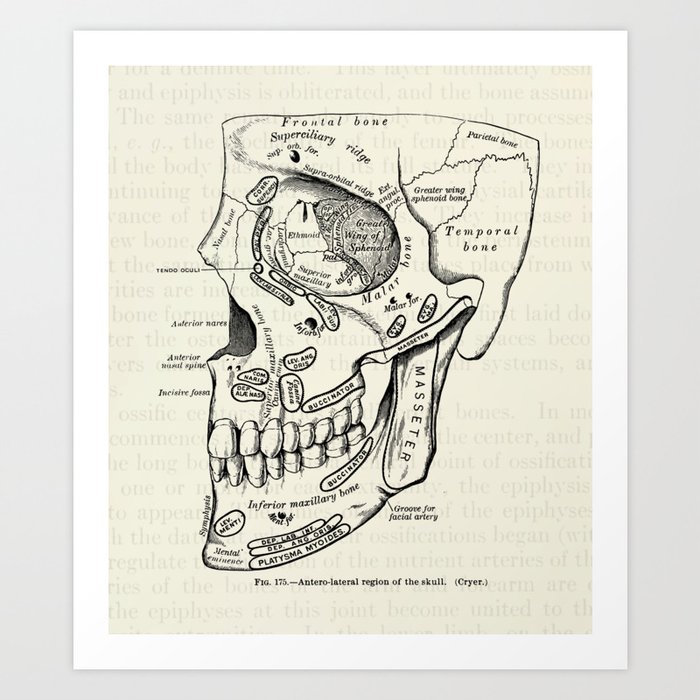The photograph is a squared image featuring a digitally edited poster on a solid gray wall. The rectangular poster, with a large thick white border, displays an illustration reminiscent of an old textbook page. The background of the poster is a tan color, designed to evoke the appearance of aged paper with semi-transparent gray text scattered across it. 

At the center of the poster is a detailed, grayscale drawing of the left side of a human skull, partially presented, from just above the eyebrow to the jaw. The skull illustration includes various labels indicating different anatomical parts, such as the "temporal bone" on the right side, the "frontal bone" at the top, and other labeled sections like the "great wing". The meticulous black ink lines and shading underscore the informative, diagram-like nature of the drawing, with several annotations in Latin around features such as the eye socket, jaw, and nasal bones. The deliberate cracks and details add to the vintage, scholarly atmosphere of the piece. A subtle shadow surrounds every edge of the poster, emphasizing its digitally imposed presence on the gray background.